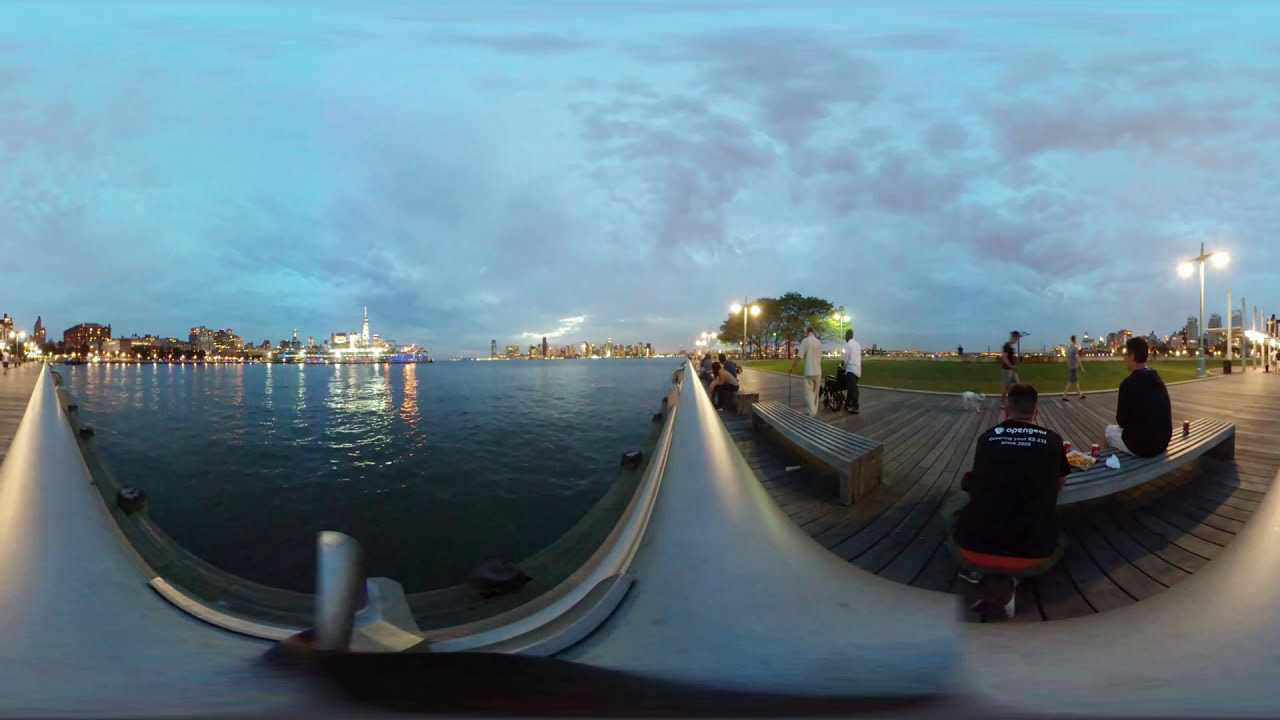The image captures a serene water scene at dusk, showcasing a picturesque combination of natural and urban elements. The sky, a blend of blue and purple hues, stretches across the horizon, partially obscured by clouds. On the left side of the image, a body of water mirrors the lights and silhouettes of well-lit buildings on the distant shoreline. Reflections dance on the water’s surface, adding a layer of tranquility to the scene. 

The central portion reveals a cement walkway extending into the horizon, splitting the scene into two distinct areas. To the right of the walkway lies a charming wooden boardwalk, curving gently along the waterline. Numerous wooden benches line this boardwalk, where people sit leisurely, some enjoying drinks and snacks, while others walk by, including a couple of individuals pushing a wheelchair and walking pets. Green patches add a touch of nature to this inviting space. 

Further along the boardwalk, a few large trees stand tall, enhancing the scenic beauty. The right half of the image, dominated by the warm activities of people in the evening light, contrasts with the serene, reflective left half, creating a harmonious blend of lively human activity and peaceful natural backdrop. The scene’s wide-angle perspective gives an immersive view, capturing not only the immediate surroundings but also the broader cityscape that lies beyond the water, making it a vibrant yet tranquil depiction of dusk by the waterfront.